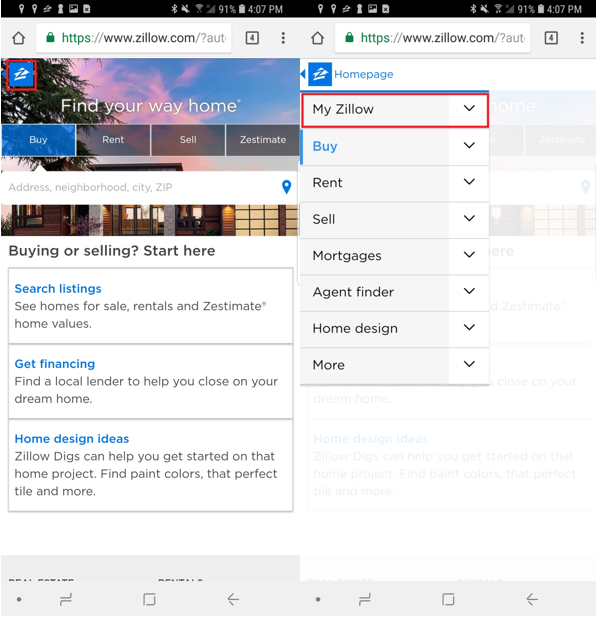The image comprises two smartphone screenshots stitched together, evident from the dual Google Map notifications at the top. The upper portion of the screen is cluttered with multiple notifications: two Google Map pins, an SD card symbol, a keyhole icon, and a screenshot indicator. Additionally, there's a pie chart notification, Bluetooth symbol, and a muted sound icon. A Wi-Fi indicator reflects connectivity, though the signal bar shows no cell service. The battery is at 91%, and the time displayed is 4:07 PM.

A dark grey bezel at the top contains a house silhouette, a secure URL marked by a green lock, and the text "HTTPS://www.zilla.com/?AUT". Below it, a black square with the number "4" and three ellipses indicate further options.

The central part of the image captures an interface with a background sky in shades of dark blue and pink, alongside a dark green tree on the left. Foreground elements include a blue box with a white up arrow framed in red, and the bold white text "Find your way home."

Below this header, there are interactive buttons: the "Buy" button is selected in blue, followed by "Rent" in a semi-transparent black, then "Sell" and "Zestimate" (spelled out). A white rectangle contains the placeholder text "address, neighborhood, city, ZIP" in grey, accompanied by a blue pin icon. Outside this field, dark grey text reads "Buying or selling? Start here."

Three major clickable rectangles with dark grey borders offer further actions:
1. "Search Listings" in bold blue, with a grey description: "See homes for sale, retailers, and Zestimate home values."
2. "Get Financing" in bold blue, alongside a grey note: "Find a local lender to help you close on your dream home."
3. "Home Design Ideas" in bold blue with a grey detail: "Zillow Digs can help you get started on that home project."

To the right, an opaque background overlays additional navigation features. The Zillow logo is next to the italicized blue text "Home Page." Below it, a dropdown menu reveals options, of which "My Zillow" is selected in red. Continuing the list, "Buy" is highlighted in blue, followed by "Rent," "Sell," "Mortgages," "Agent Finder," "Home Design," and "More," each having grey backgrounds and dropdown arrows.